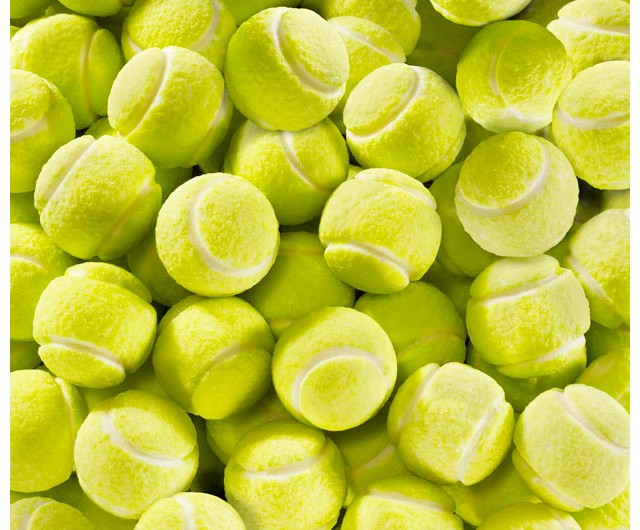This image shows an overhead view of numerous greenish-yellow tennis balls, stacked and densely packed together, covering the entire frame from corner to corner. Each tennis ball features the standard distinctive design of a tennis ball with two white curved grooves running across their surface, segmenting the balls into hemispheres. The shading on the balls appears inconsistent, making the image seem less lifelike. The arrangement is such that the balls are oriented in various directions, filling the picture with layers of tennis balls extending from the top to the bottom and stretching from the left side to the right side of the image. The depth and density of the stacking suggest there are approximately 50 balls in the frame, with some appearing closer to the viewer while others recede into the background.